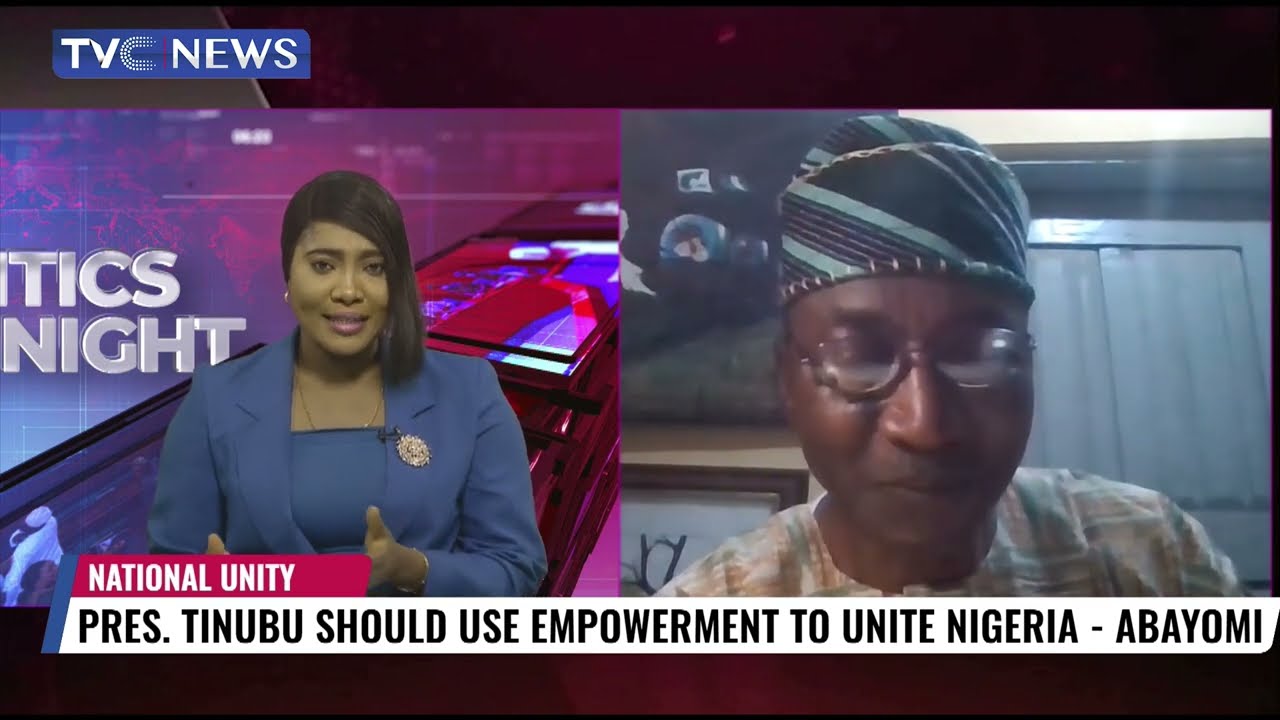This image depicts a nightly broadcast from the TVC News station, as indicated by the white text in a blue banner in the upper left corner. The split-screen format shows two individuals: the news anchor on the left and an interviewee on the right. The news anchor, a dark-skinned woman with shoulder-length black hair partially covering her face, is dressed in a coordinated blue suit jacket and undershirt. Her attire features a gold-colored badge on the right side of her chest, a thin necklace, and earrings. Her lips are light pink, and her mouth is slightly open. Behind her, partial graphics display the words "POLITICS NIGHT" in silver letters. A white banner with a ticker at the bottom reads: "National Unity - Prez Tinubu should be empowered to unite Nigeria - Eboyami."

On the right side of the screen, the interviewee, a black individual, wears glasses and a traditional Nigerian outfit, including a headwrap with diagonal lines in shades of green. Their attire suggests cultural significance, adding context to the discussion about national unity.